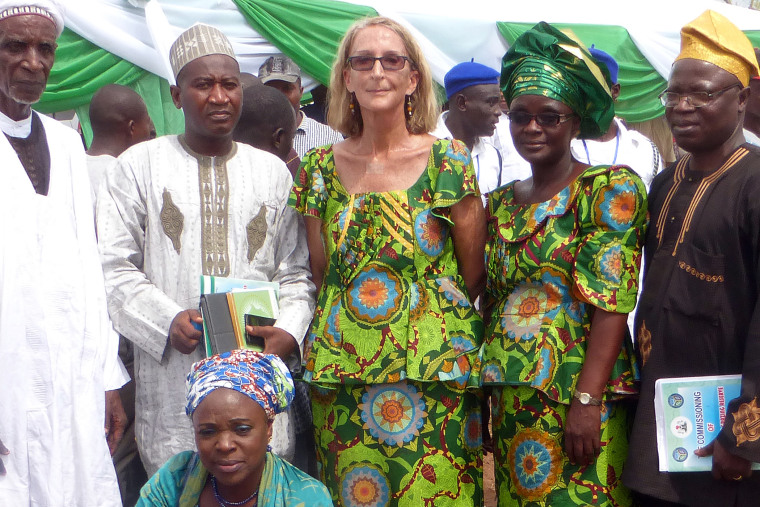The photograph captures a diverse group of individuals predominantly dressed in traditional African attire, suggesting a cultural or formal event, possibly a conference or an award ceremony. Central to the image is a white woman, notable for her presence among the predominantly black individuals surrounding her. Both she and the black woman to her left (our right) are wearing similar patterned green dresses, paired with sunglasses that add a cohesive visual symmetry. The woman to the right also sports an African-style hat, enhancing the authenticity of the attire.

Flanking the central figures are three men: one man on the right in a black shirt, and two men on the left in lighter, long shirts that extend beyond the hips. Each of these men wears a hat, contributing to the uniformity of the traditional dress code. An additional layer of visual interest is provided by a black woman crouched in front of the leftmost man, her outfit distinct with a head wrap.

In the background, a crowd mingles, adding a lively atmosphere to the scene. Notable details include the men holding booklets or paperwork, indicating an organized event. The detailed, harmonious blend of traditional garments and the intermingling of attendees in the backdrop collectively enrich the narrative of this vibrant and culturally significant gathering.